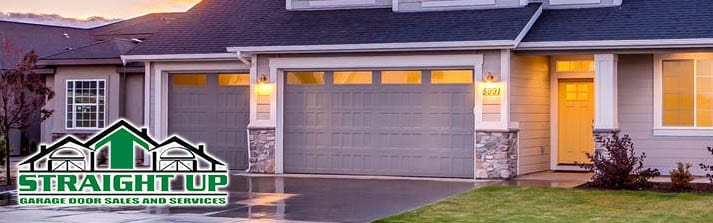In this captivating image of a suburban home, the scene is set at dusk as the sun has already begun to set, painting a serene ambiance. The house features a meticulously maintained exterior, accentuated by warm light bulbs that illuminate the surrounding area. The elegant facade includes two distinct garage doors—a larger, primary garage door and a smaller one, both seamlessly integrated into the structure. There is a centrally located door with an adjacent window on the right side, emitting a cozy glow. To the left, another window and a lush tree add a touch of natural beauty to the scene. The house is surrounded by a variety of trees and plants, enhancing the picturesque setting. The roof, with its sleek black shingles, complements the overall aesthetic of the home. Prominently displayed is a caption along with a logo for "Straight Up Garage Door Sales and Services," suggesting a focus on garage door solutions. The overall image exudes a welcoming and well-kept atmosphere, perfect for a tranquil evening.